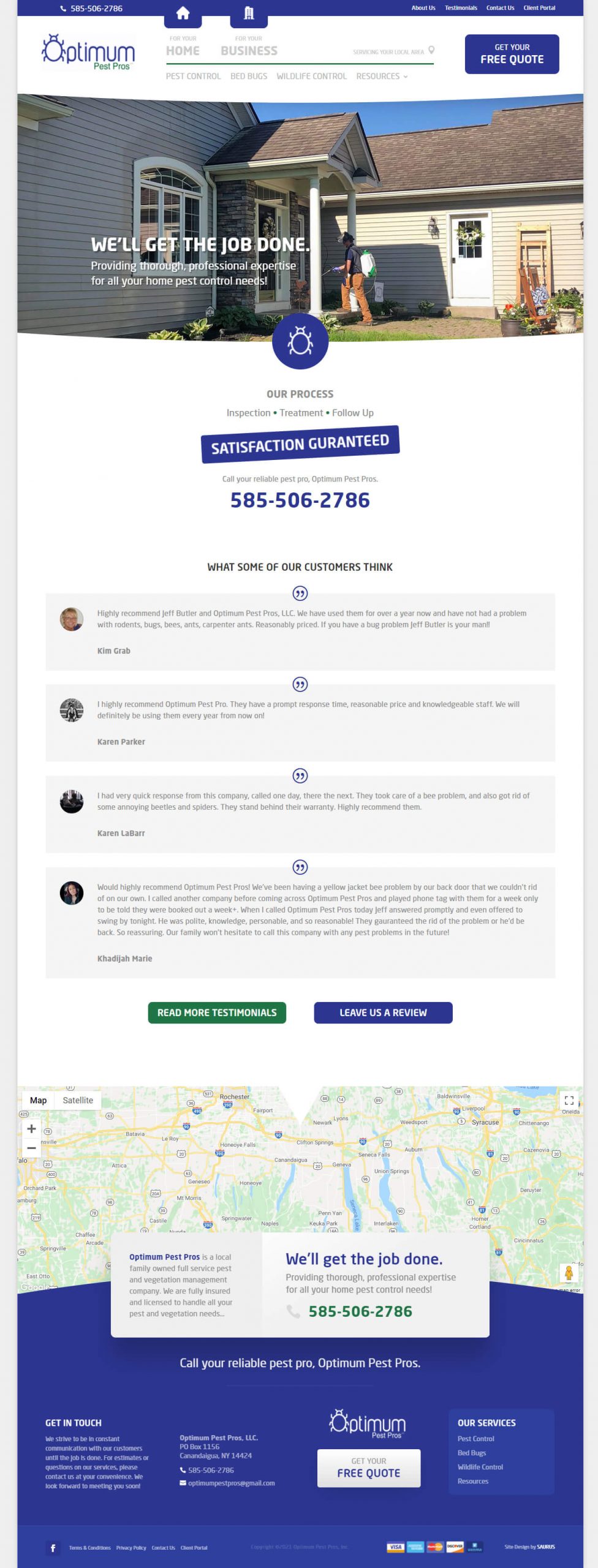Screenshot from the Optimum Pest Pros website showcasing professional home pest control services. The image captures an exterminator spraying insecticide near the front entrance of a house, emphasizing the company's on-site expertise. The site banner reads, "We'll get the job done - providing thorough professional expertise for all your home pest control needs," highlighting their commitment to quality service. 

The page features a "Satisfaction Guaranteed" box, along with a prominently displayed contact number, 585-506-2786, in blue text. A section of customer reviews is included, with a notable testimonial from Kim Grab: "Highly recommended Jeff Butler and Optimum Pest Pros LLC. We have used them for over a year now and have not had a problem with rodents, bugs, bees, ants, carpenter ants. Reasonably priced. If you have a bug problem, Jeff Butler is your man." The review includes an avatar of Kim Grab's face and is accompanied by reviews from Karen Parker, Karen Labars, and Khadijah Marie.

At the bottom of the screenshot, a map is displayed with a box containing additional information about the company, such as their location, service area, and contact details. An email address and a "Free Quote" button are also provided, guiding potential customers toward further action.